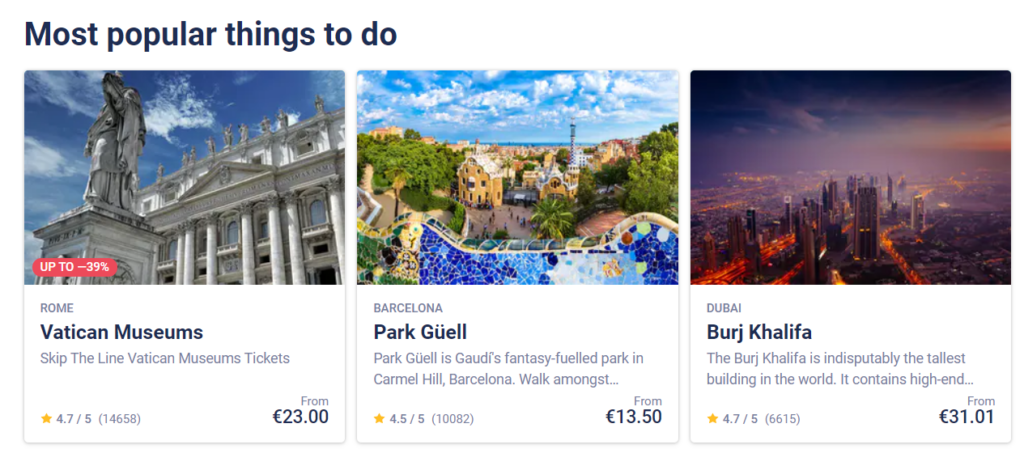**Caption:**

The image features a promotional graphic with a white background at the top and black text that reads "Most Popular Thing to Do." Below, there is a section showcasing the outside of the Vatican on a partly cloudy day. In the foreground, a statue sits atop a square-shaped pedestal in front of a building with large marble columns. On the lower left side, a red oblong box indicates "Up to 39% Off." Beneath it, more text details the offer: "Rome, Vatican Museum - Skip the Line. Vatican Museum tickets, 4.7 out of 5 stars, 14,658 reviews, starting from 23 Euros."

To the right, a second section displays an image of a charming villa amidst palm trees under a partly cloudy sky. The caption for this part reads, "Barcelona, Parc Güell - Parc Güell is Gaudí's Fantasy-Filled Park on Carmel Hill, Barcelona. Walk Amongst, 4.5 out of 5 stars, 10,082 reviews, from 13.50 Euros."